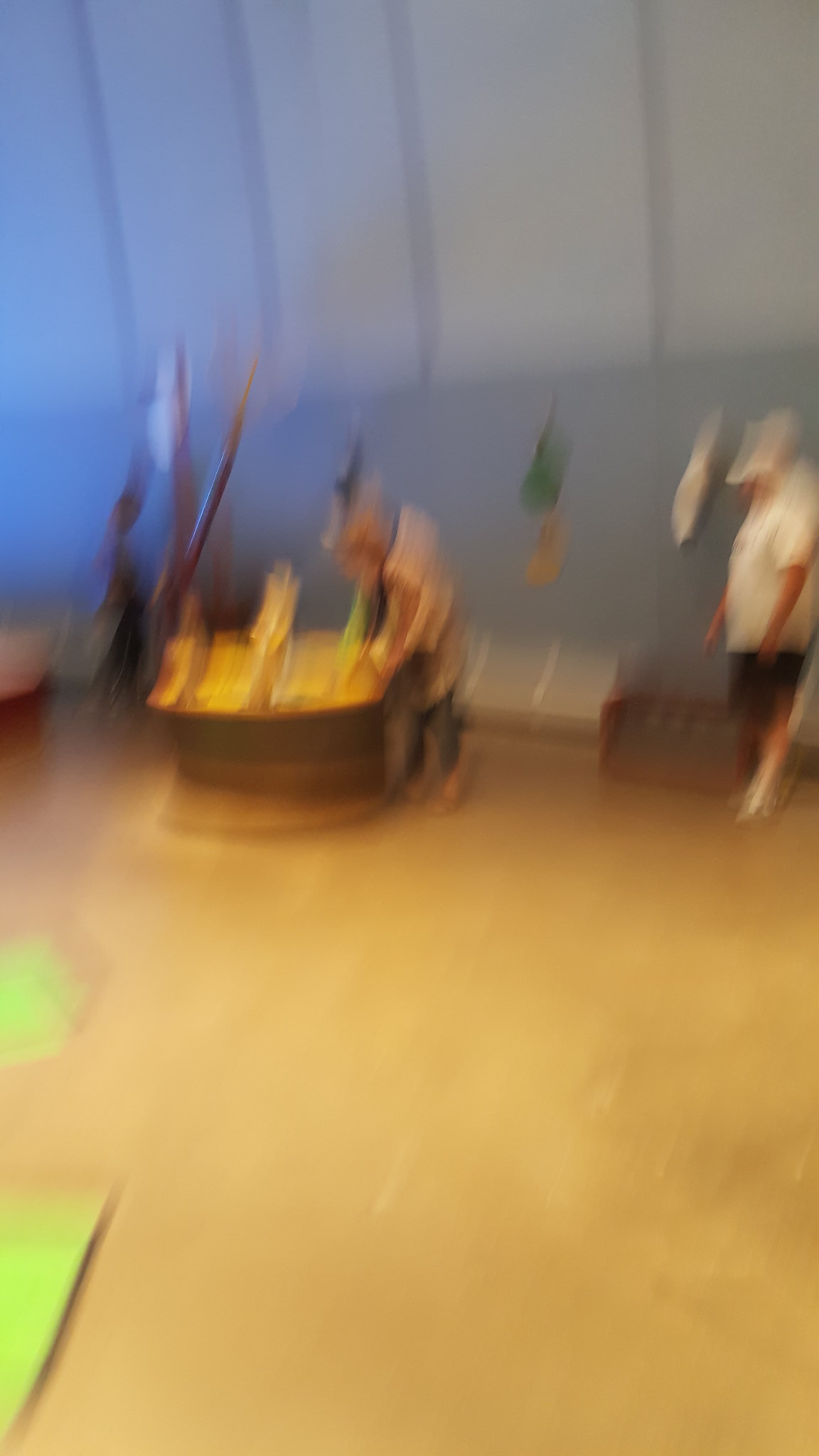The image depicts a bustling, blurred outdoor scene on a stone ground. Prominently on the bottom left and along the left side are vivid yellow areas. A sloped rooftop is visible towards the left side of the frame. Black lines intersect with a mixture of white and green hues towards the bottom. Mid-right in the image is a man with notable features: a large mouth, wearing a white cap, white shirt, black shorts, and white shoes. Behind him, there is a patch of green.

To his left, there's another person, possibly engaged in an activity involving shirts, who seems to be in motion. This individual is clothed in gray pants and brown shoes, appearing to look down at a table. Further to the left, there seems to be an oversized pen leaning over another table. The background is characterized by a circular formation with an overall light blue tone and scattered white benches, creating an aesthetically pleasing array.